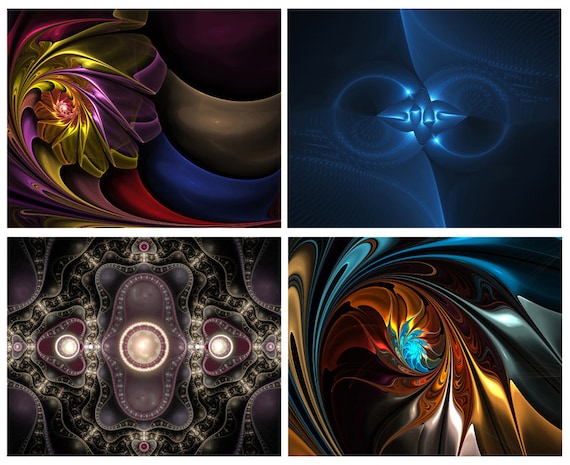This image contains a collage of four vividly colorful and abstract digital artworks. Each piece is presented in a grid formation against a single background.

- **Top Left Image**: This artwork features swirling, vivid colors of purple, green, and gold. The design resembles a spinning wheel or an ocean wave in wild colors, with suggestions of a swirling bowl and flowing ribbons in shades of copper, blue, and fluorescent yellow.

- **Top Right Image**: This design predominantly showcases hues of blue with a dark blue background. Central to the piece are three interlocking round objects in light blue and white, creating a laser light effect with a glowing centerpiece.

- **Bottom Left Image**: This piece is a kaleidoscopic design highlighted by purples, blacks, and browns, resembling the intricate and repetitive patterns seen inside a kaleidoscope. Colors used include gold, red, and yellow, creating a rich and mesmerizing visual.

- **Bottom Right Image**: The final artwork features dynamic swirls of paint converging towards a star in the center. The design also includes a tube-like form inside the swirling pattern, using colors like green, gold, and yellow to create a sense of depth and motion.

Together, these four images present a captivating and abstract exploration of shapes, colors, and patterns.